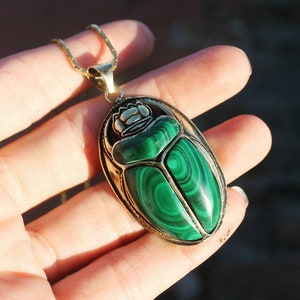The image is a square format photograph capturing a close-up of a left hand, displaying its four fingers and part of the palm against an entirely black background. Draped elegantly across the fingers is a necklace made of a gold chain, extending over the index finger. The focal point of the photograph is a large, ornate scarab beetle pendant, occupying the width of the bottom three fingers. This pendant is an oval-shaped piece of jewelry, surrounded by intricate gold detailing. The scarab's wings and body are adorned with vibrant emerald-green stones, interspersed with lighter green and black swirls, resembling malachite. The head of the scarab is crafted in silver with additional silver details giving it a distinct beetle-like appearance. This elaborate pendant suggests a significant piece of statement or costume jewelry, with its craftsmanship hinting at a possibly Native American influence.